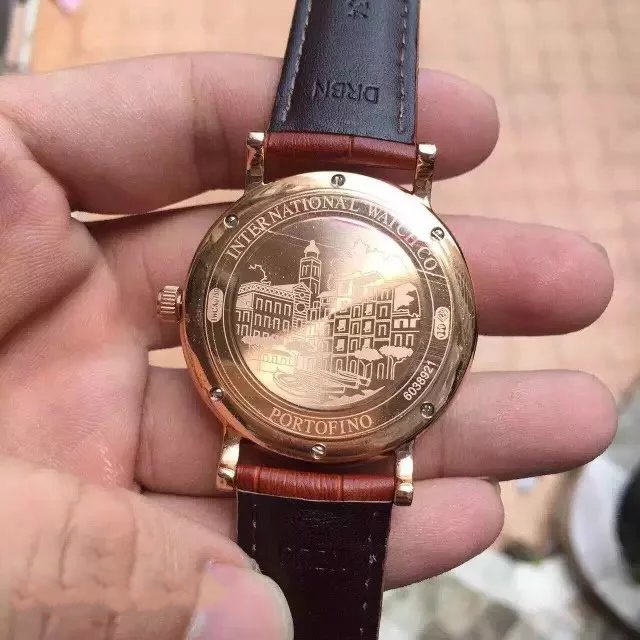In the photograph, a close-up captures the right hand of a person with white skin, palm up, thumb positioned at the bottom of the image. The hand is holding a luxurious, large-sized wristwatch with an intricate design. The watch boasts a black leather band with visible stitching and a slim, contrasting reddish-brown leather border where it attaches to the gold watch case. The gold face of the watch features an etching of a building in the center. Above this etching, the words "International Watch Company" are inscribed, while "Portofino" is engraved below. Flanking these engravings to the right is a serial number and other identifying marks in an oblong shape. The watch, which includes various screws and a winding knob on the left side, possibly has diamonds inset in the gold case representing the numbers on the clock. The background of the image is a blurry peachy mauve color, providing a contrast that makes the details of the watch and hand stand out.